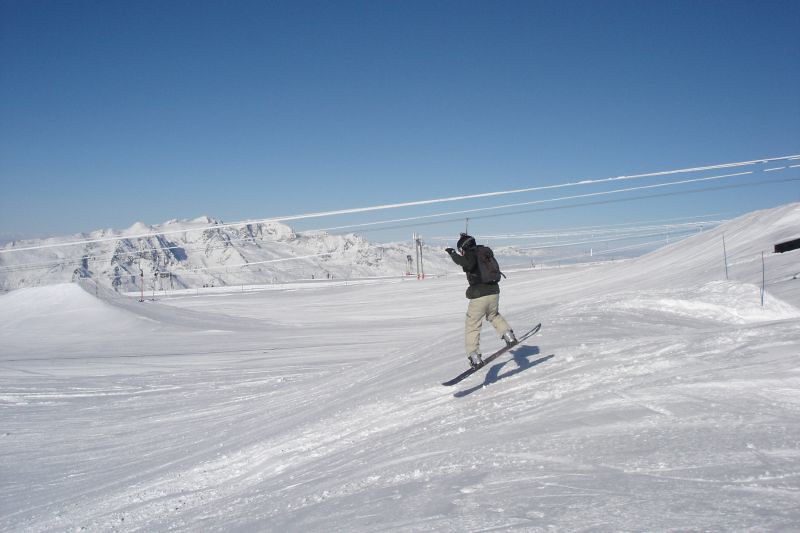This image captures a thrilling moment of a lone snowboarder mid-air, gliding down a gentle, snow-covered slope from right to left. The snowboarder, who appears to be around one to two feet above the ground, is equipped with a black helmet, potentially adorned with a GoPro camera, and is wearing a black backpack, a black jacket, and beige pants. They sport silvery snow boots and black gloves. A black snowboard supports their flight against a backdrop of a clear, bright blue sky. Suspended cables, likely part of a ski lift, draped in snow and stretching across the scene, refine the setting of this remote, pristine winter landscape. Distant, snow-capped mountain tops frame the scene, adding depth and grandeur to the action shot. The snowboarder’s dynamic stance, with one hand raised near their face, and their shadow cast crisply on the snow beneath, highlight the bright and vivid day on the slopes.